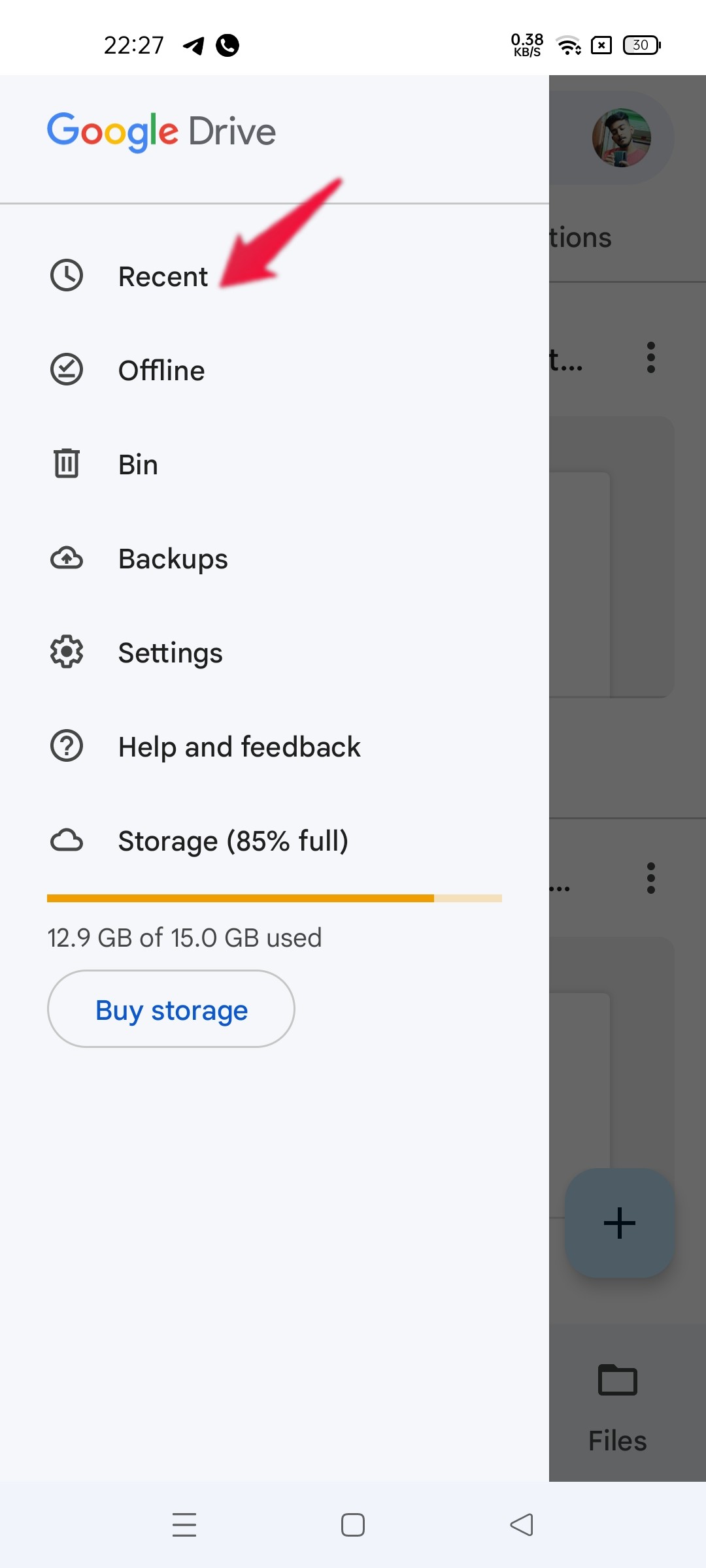This is a screenshot taken on a phone displaying the Google Drive app's interface. At the very top, there's a white status bar. On the upper left corner of this bar, a time stamp reads "22:27." Moving rightward, there is a location services icon followed by a small telephone symbol. In the upper right corner, the status bar also shows the battery percentage, Wi-Fi signal strength, and other icon elements that are too small to discern clearly. 

Below the status bar, the Google Drive logo is prominently displayed; "Google" is written in the signature multi-colored letters, and "Drive" is in black. Underneath this logo, the sidebar menu contains the following options listed vertically: Recent, Offline, Bin, Backups, Settings, Help and Feedback, and Storage with an 85% usage indicator. The storage indicator is represented by an orangish-yellow line, filling up to 85%, signifying 12.9 GB of 15.0 GB used. Beneath this indicator, there's a blue button labeled "Buy storage."

Notably, a red arrow on the screenshot points directly to the "Recent" option in the sidebar menu, emphasizing that selection.